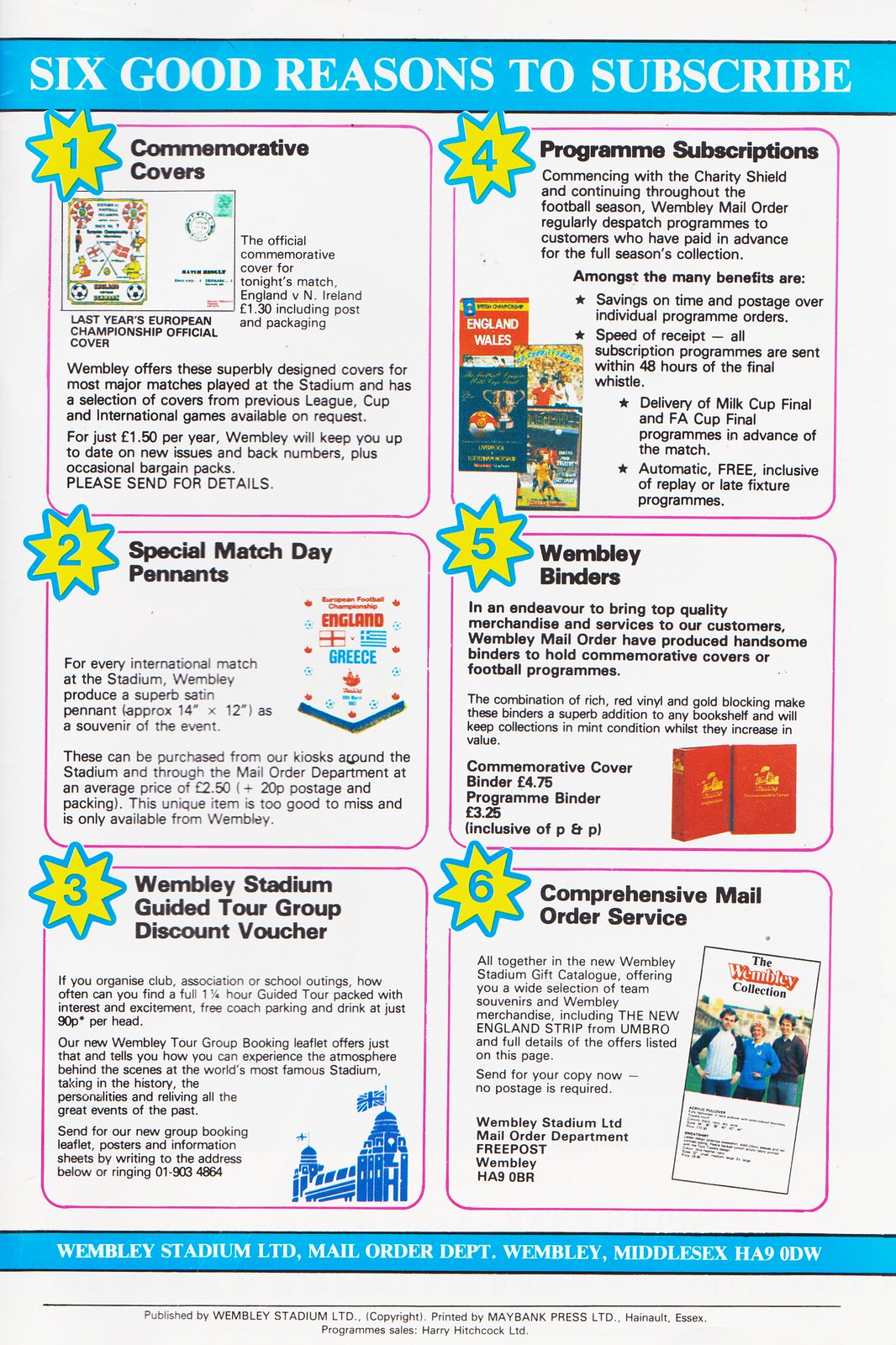This image is a detailed page from a magazine with a white background, prominently featuring a light blue stripe across the top. Inside the stripe, "Six Good Reasons to Subscribe" is displayed in bold white lettering. Below this header, the page is sectioned into three rows of two boxes each, creating a total of six framed rectangles. Each rectangle has the same white backdrop and contains a reason to subscribe, marked by yellow starbursts outlined in blue, sequentially numbered one through six in blue font.

In the first box on the upper left, labeled number one, the caption reads "Commemorative Covers" in black text. Directly below it, reason number two is "Special Match Day Pennants," accompanied by an illustration of a pennant. Reason number three, located in the upper right box, states "Wembley Stadium Guided Tour Group Discount Voucher." 

The next column continues with box four labeled "Program Subscriptions,” showcasing the benefits of subscribing to regular football programs. Reason five, "Wembley Binders," is presented in the subsequent box, featuring visuals of the binders. Finally, box six explains the "Comprehensive Mail Order Service" and depicts related flyers.

Along the bottom of the page, another blue stripe runs across, bearing additional information in white text: "Wembley Stadium LTD Mail Order Department, Wembley, Middlesex HA90DW." This indicates the magazine’s publisher and contact address for mail orders, emphasizing the dedicated service provided to subscribers.